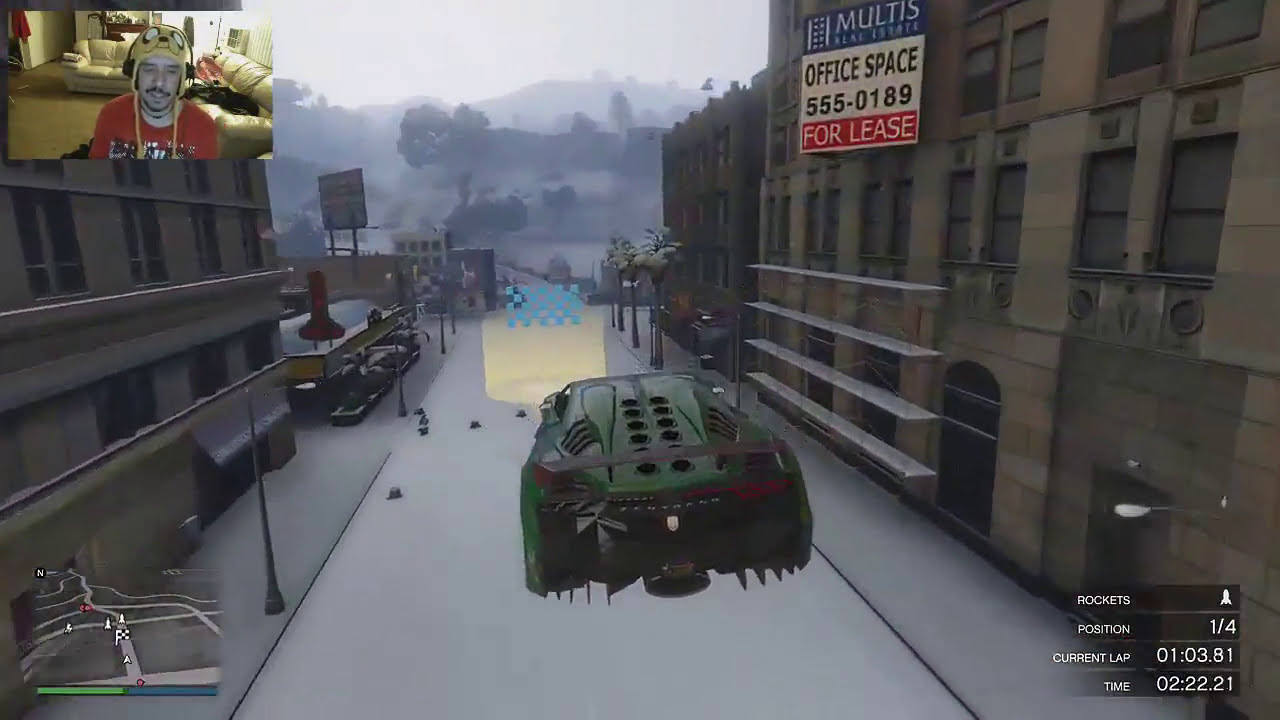The image captures a scene from a futuristic video game, centrally featuring a green hovercraft navigating down a city street amidst a foggy and misty atmosphere suggestive of ongoing warfare in the distance. On the right side of the hovercraft, a four or five-story building bears a sign that reads "Maltese Office Space 555-0189" with a red "for lease" box underneath. To the left, another building stands in view. In the upper left corner, a live stream overlay displays a man with a mustache, wearing a yellow hat and headphones, likely the player or streamer of the game. Below him, a map of the race track is visible in the bottom left, guiding the hovercraft's direction. In the bottom right corner, game stats are shown, indicating "Rockets," positioned "one out of four," with lap and time details "103.81" and "222.21." The colors in the image are varied, including red, yellow, brown, white, blue, light blue, and green, providing a vibrant and dynamic visual experience.